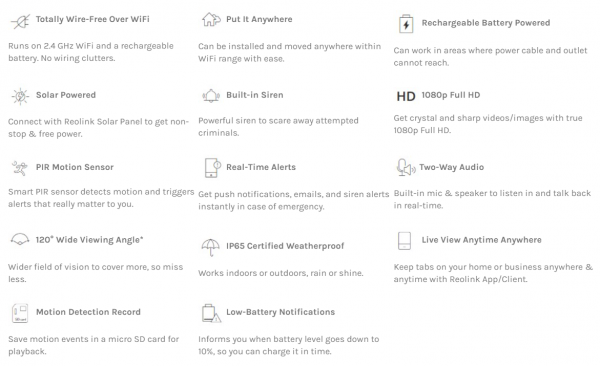**Descriptive Caption:**

The image features a comprehensive promotional infographic on a pristine white background, detailing the standout features of a security device. 

On the top left, all the headings are in gray. The first section reads, "Totally Wire-Free Over Wi-Fi," indicating that the device operates on 2.4 GHz Wi-Fi and a rechargeable battery, ensuring no writing clutters. Below, "Solar Powered" highlights the ability to connect with the Reolink solar panel for non-stop, free power. 

Next, "PIR Motion Sensors" elaborates that a smart PIR sensor detects motion and triggers important alerts. Adjacent to it, "120° Wide Viewing Angle" emphasizes a wide field of vision, ensuring fewer missed details. Then, "Motion Detection Record" explains that motion events are saved on a micro SD card for playback, with gray icons accompanying each point.

At the center, bold text declares, "Put it Anywhere," explaining that the device can be installed and moved anywhere within Wi-Fi range effortlessly. Additional features highlighted include:

- "Built-in Siren" for scaring away potential criminals with a powerful alarm.
- "Real-Time Alerts" for instant push notifications, emails, and siren alerts in emergencies.
- "IP65 Certified Weatherproof" ensuring the device works indoors or outdoors in varying weather conditions.
- "Low Battery Notifications" that alert users when battery levels drop to 10%, prompting timely recharge.

On the top right, "Rechargeable Battery Powered" states that the device can operate in areas without power cable access. In bold black, "HD," followed by gray text, highlights "1080p Full HD," ensuring crystal-clear videos and images. Accompanying features include:

- "Two-Way Audio" with a built-in mic and speaker for real-time listening and talking.
- "Live View Anytime, Anywhere" allowing monitoring of home or business through the Reolink app-client from any location.

Overall, the image meticulously outlines the device’s extensive features, emphasizing versatility, ease of use, and robust security measures.